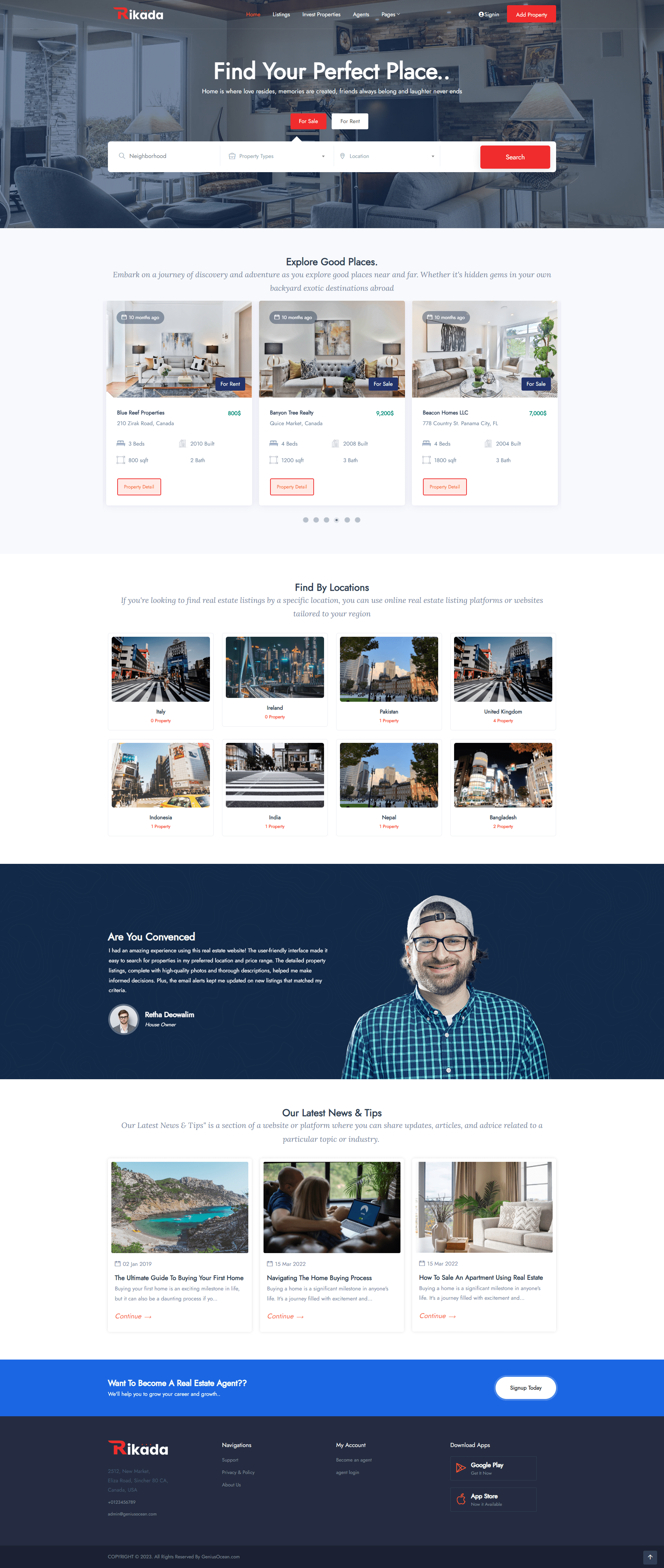**Screenshot Description of Rikada's Website**

This screenshot showcases the homepage of a website called Rikada, identifiable by its distinctive logo where the "R" is colored in red followed by "IKADA" in black. The top navigation bar includes options for 'Home,' 'Listings,' 'Properties,' 'Agents,' and 'Pages,' along with a 'Sign-In' option. There's a prominently placed red button labeled 'Add Property.'

The central section of the page features the website's main advertisement banner with the headline, "Find Your Perfect Place." Beneath it, users are prompted to search for properties either for sale or for rent. The search functionality allows filtering by neighborhood, property types, and specific locations, all accessible via a search bar. The background image of this section depicts a stylish living room.

Below the main banner, there's a section titled "Explore Good Places," highlighting three featured properties listed by Blue Leaf Properties, Banyan Tree Realty, and Bacon Homes, LLC. Notably, one property priced at $9,200 per month is mentioned, indicating a high rental cost.

Further down, there's a "Find by Location" section, displaying the geographic areas served by Rikada. The availability of properties is limited, with listings including:
- 1 Property in Pakistan
- 4 Properties in the United Kingdom
- 2 Properties in Bangladesh
- 1 Property in Nepal
- 1 Property in India
- 0 Properties in Italy
- 0 Properties in Ireland

A notable visual element features a person resembling a casual individual—wearing a cap, sporting a beard, and dressed in a casual shirt—under a heading presumably questioning user concerns. The screenshot also hints at numerous hard-to-read menu options at the bottom of the page.